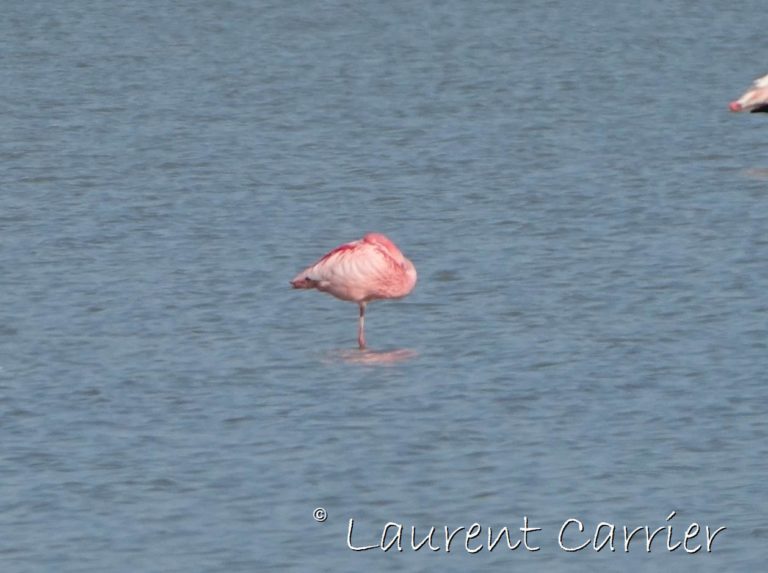This photograph captures a serene, shallow body of water with only slight ripples and a gradient of blue from deeper at the top to lighter at the bottom. The focus of the image is a pink flamingo standing on one foot in the center, with its head tucked behind its wing, making it invisible. The flamingo showcases a spectrum of pink tones: almost red along its back, light pink on its wings, and darker pink on its belly. Its feet are submerged, casting subtle shadows beneath. In the top right corner, the tail end of another flamingo is partially visible. The photograph is marked with large, white lettering at the bottom reading, "copyright, Laurent Carrier (L-A-U-R-E-N-T, C-A-R-R-I-E-R)."